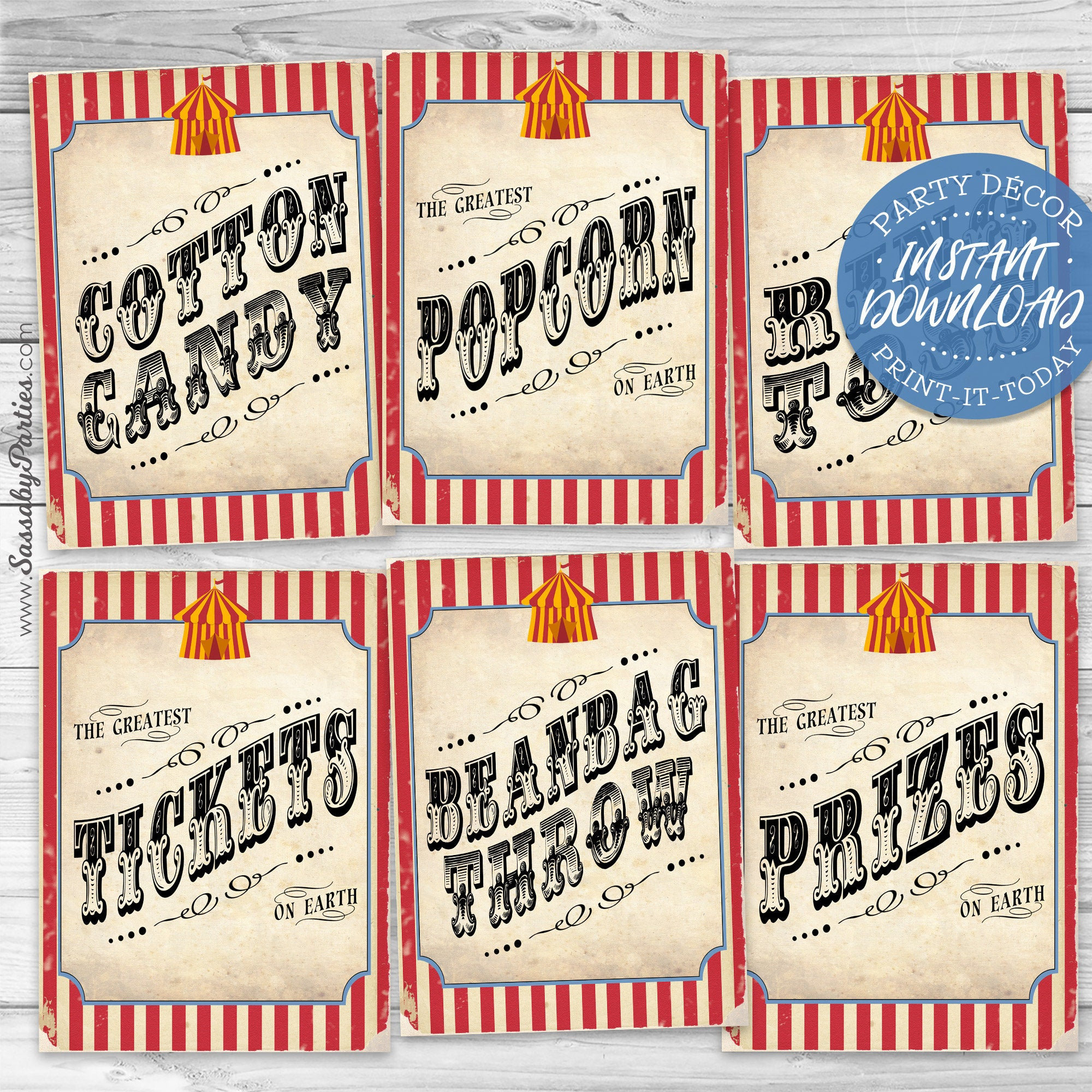The promotional image showcases an array of six colorful, vintage circus-themed printable posters arranged in two rows of three against a light gray wooden surface. Each poster features a vibrant red and white striped border, encasing a cream-colored panel adorned with a classic circus tent motif at the top. Bold black text on each panel denotes various circus attractions, reading from left to right: "Cotton Candy," "The Greatest Popcorn on Earth," and an obscured title beneath a semi-transparent blue circle on the first row. The second row displays "The Greatest Tickets on Earth," "Bean Bag Throw," and "The Greatest Prizes on Earth." The semi-transparent blue circle in the top right corner bears white text advertising "Party Decor, Instant Download, Print It Today." Complementing the layout, the website URL www.sasbyparties.com is vertically aligned along the left edge of the image, emphasizing a sleek and organized presentation.